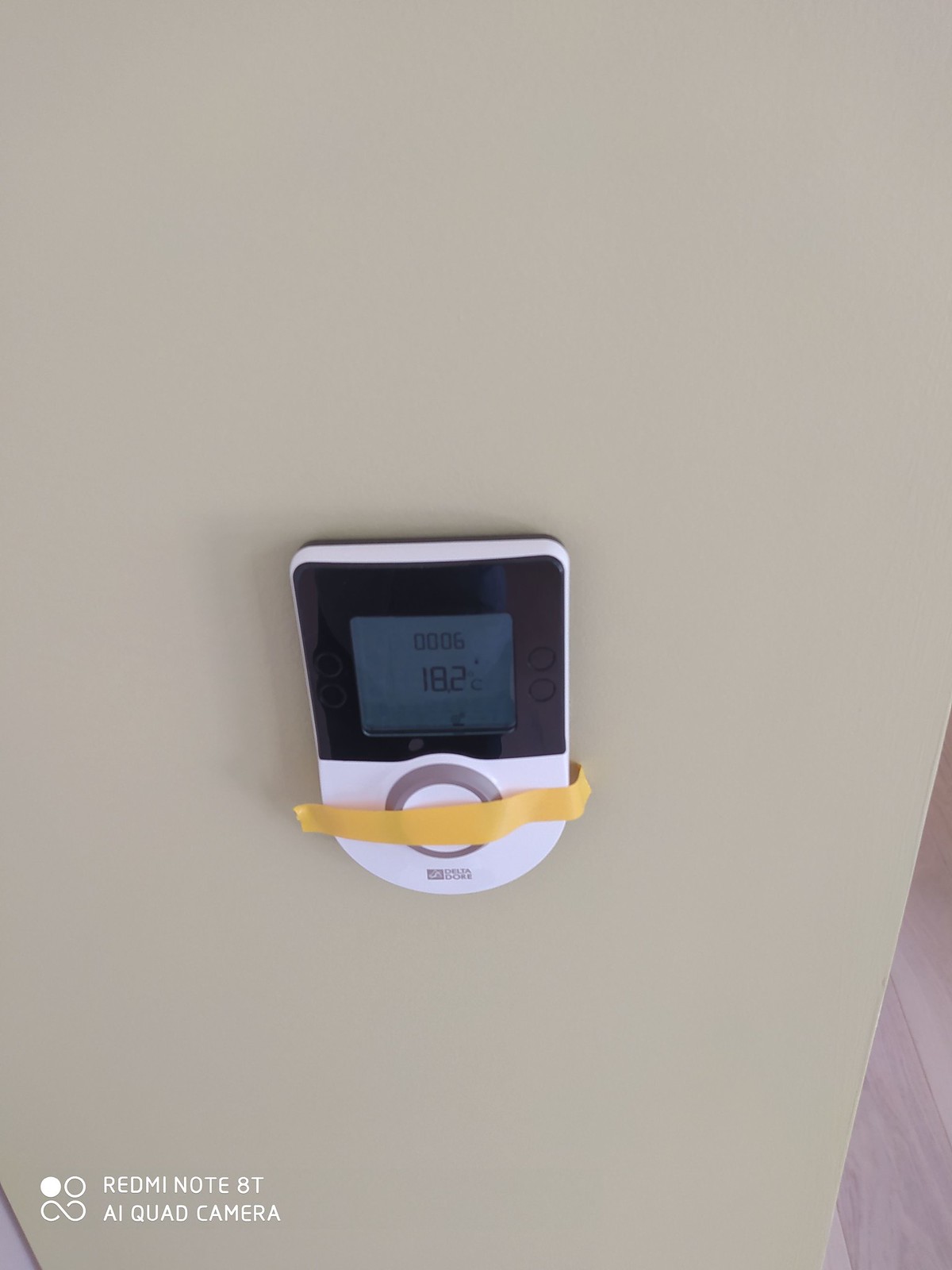The image features a thermostat mounted on an off-white, slightly tan wall. The edge of the wall is visible, with light wood flooring seen below. The thermostat is partially covered by a piece of tape that extends from the front to behind the device. It has a unique shape: squared at the top and rounded at the bottom. The lower half of the thermostat is white and includes a gray circle with a smaller white circle inside it, along with symbols resembling the Greek letter delta. The upper section is black, featuring a digital screen with two buttons on each side. The display reads 18.2 degrees Celsius, with the number 0006 positioned above it. In the bottom left corner of the screen, there are three icons: a filled white circle, an outlined white circle, and an infinity symbol, all rendered in white. The text "Redmi Note 8T AI Quad Camera" is also inscribed in white. The overall ambiance is clean and modern, subtly accented by the interplay of the wall's neutral tone and the sleek design of the thermostat.